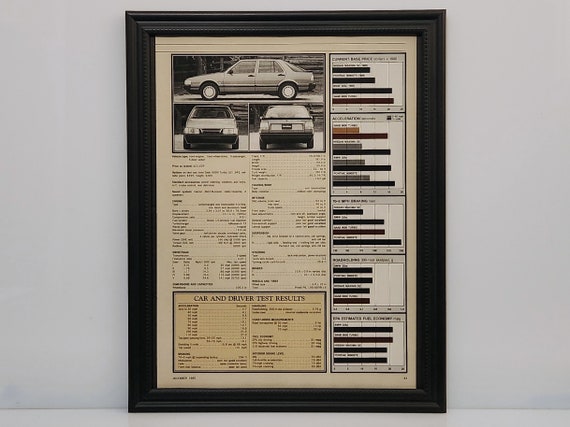This framed image features a black-and-white depiction of a likely 1980s or 1990s sedan car, viewed from the side, front, and back. The frame is black, set against a white background, hanging either in a white or blue room. On the right side of the frame, there are five color-coded bar graphs in blue, red, yellow, orange, and potentially black hues, representing various test data, though the text within them is too small to read clearly. Below the car images is an orange text box labeled "Car and Driver Test Results" in black lettering, which presumably contains specific test data and statistics about the car and driver performance. Additional text above the box likely provides further details but is also too small to be legible. The framing gives a comprehensive look at the vehicle's test results, juxtaposed with multiple views and analytical data, all encased in a sleek black wooden frame.